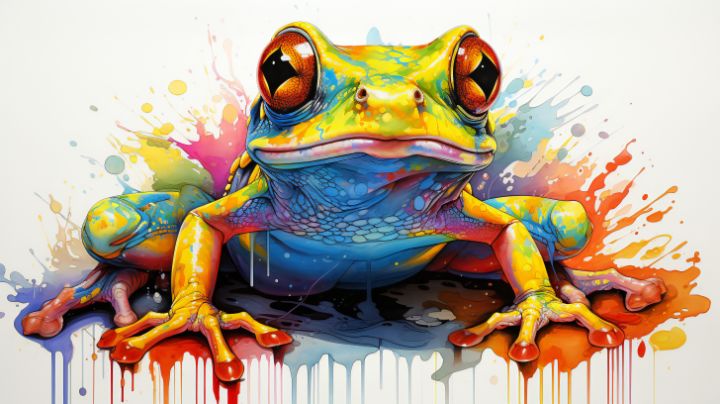This artwork features a highly detailed, psychedelic frog rendered in a digitally processed watercolor style, set against a plain white background. The frog boasts a vibrant palette of colors, with its main body being a yellowish-green hue. Its head, speckled with yellow, features big, expressive eyes that have gold and brown tones with diamond-shaped pupils. The intricate details extend to the nose, which is yellow with a touch of blue, and to the lower lip, which is an enchanting mix of blue and pink adorned with mermaid-like scales. The frog's limbs are a medley of colors: arms are painted yellow with striking red fingernails, while the legs blend yellow and orange hues with blue accents, dotted with orange swirls and large splotches of pink, blue, orange, and green paint that creatively drip down the page. The artistic use of color gives the frog a surreal quality, further emphasizing its psychedelic appearance while maintaining a realistic texture often seen in watercolor paintings.